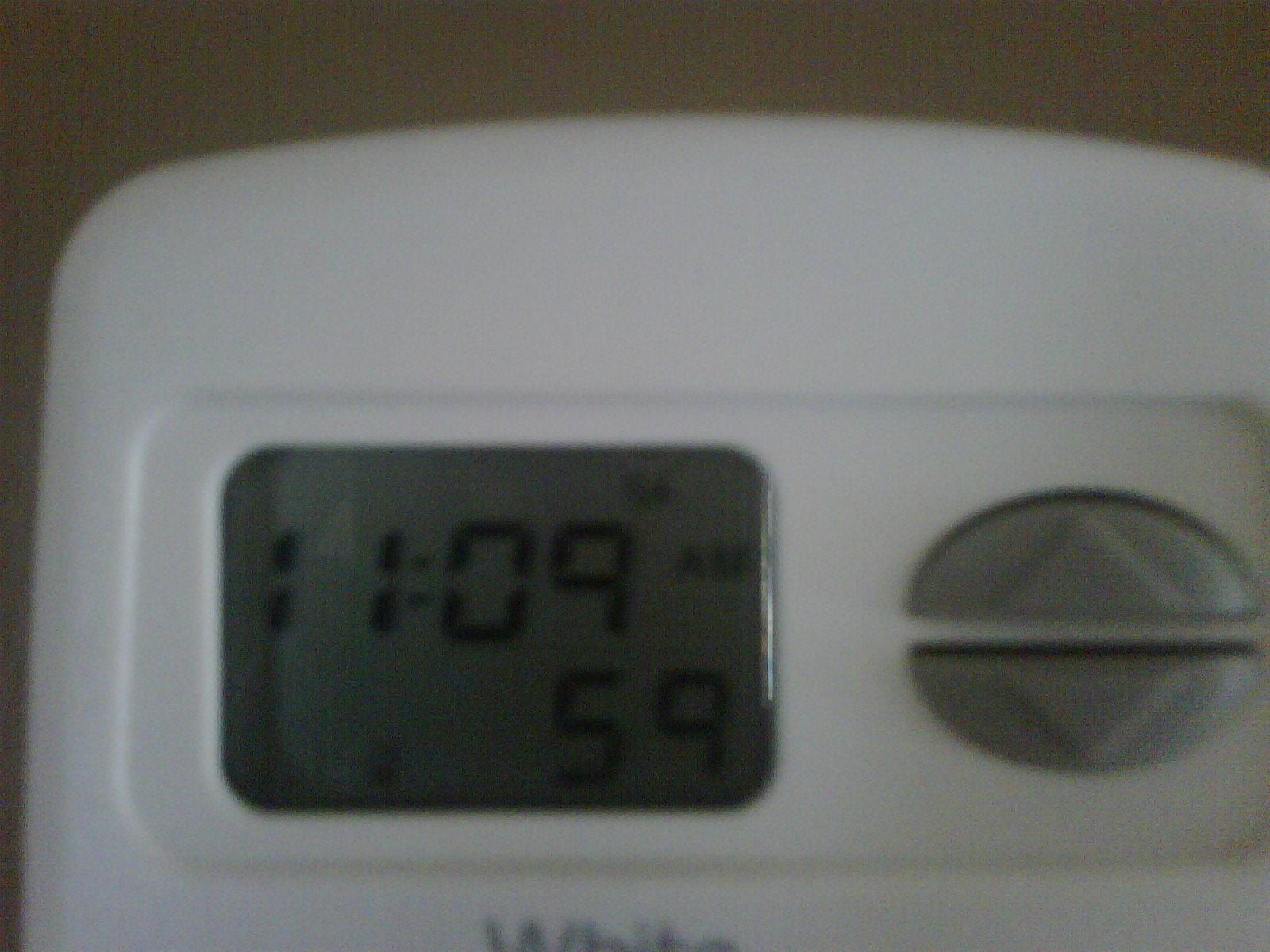The image is a close-up of a white electronic device, which appears to be either a timer or a thermostat. On the top left of the device, there is a small rectangular display screen. The screen shows the current time, "11:09," and next to the time, slightly to the upper right, the letters "A.M." can be seen. Below the time, the number "59" is displayed. The clarity of the display is somewhat compromised, making it slightly blurry. To the right of the display screen, there are two buttons arranged vertically. These buttons are shaped like a circle that has been split in half. The top half of the button features an upward-pointing arrow, indicating an increase or up function, while the bottom half of the button has a downward-pointing arrow, indicating a decrease or down function. At the very bottom edge of the device, partially cut off in the image, there is a word that is not entirely visible.